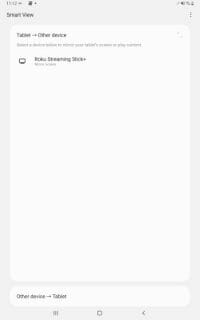The screenshot depicts a blurred settings page on an Android device with a light grey background and a lighter grey inner rectangle. At the top, there are typical phone icons including what appears to be the time. The title "Smart View" is somewhat legible. Below the title, there is a box that seems to mention a "Tablet" and possibly states "Offline device," but the text is difficult to read. Further down, another section references a device setup, displaying what looks like a little screen icon accompanied by text, possibly "Streaming Stick Plus." The screen has extensive blank space below this information. At the very bottom, there are standard Android navigation icons: three horizontal lines representing the app drawer, a square symbolizing the home button, and an arrow indicating the back button.